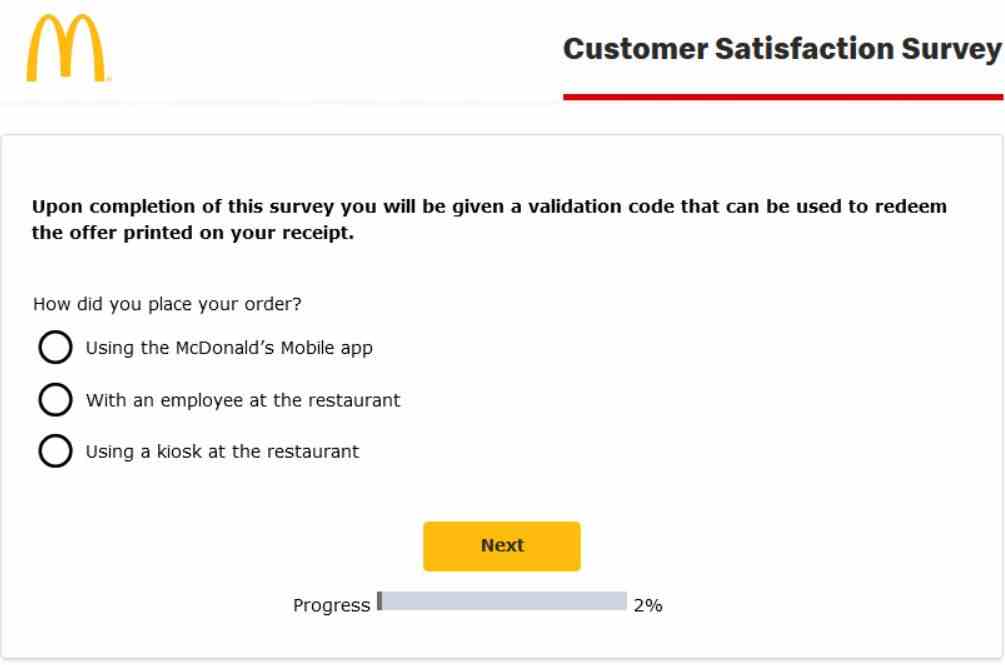Caption: 

An image displays a McDonald's customer satisfaction survey interface. In the top-left corner, the iconic McDonald's golden arches logo is prominently visible. Directly to the right of the logo, the title "Customer Satisfaction Survey" is underlined in red. Below this header, a main body of text explains the survey process: "Upon completion of this survey, you will be given a validation code that can be used to redeem the offer printed on your receipt."

Further down, the survey asks, "How did you place your order?" followed by three vertical options represented by radio buttons. The first option, "Using the McDonald's mobile app," is positioned to the right of the top button. The second option, "With an employee at the restaurant," is listed below, and the third option, "Using a kiosk at the restaurant," follows. 

Towards the bottom, a yellow "Next" button invites participants to proceed with the survey. A progress bar below the button shows minimal progression, indicating that the survey is just beginning, marked at around 2% completion.